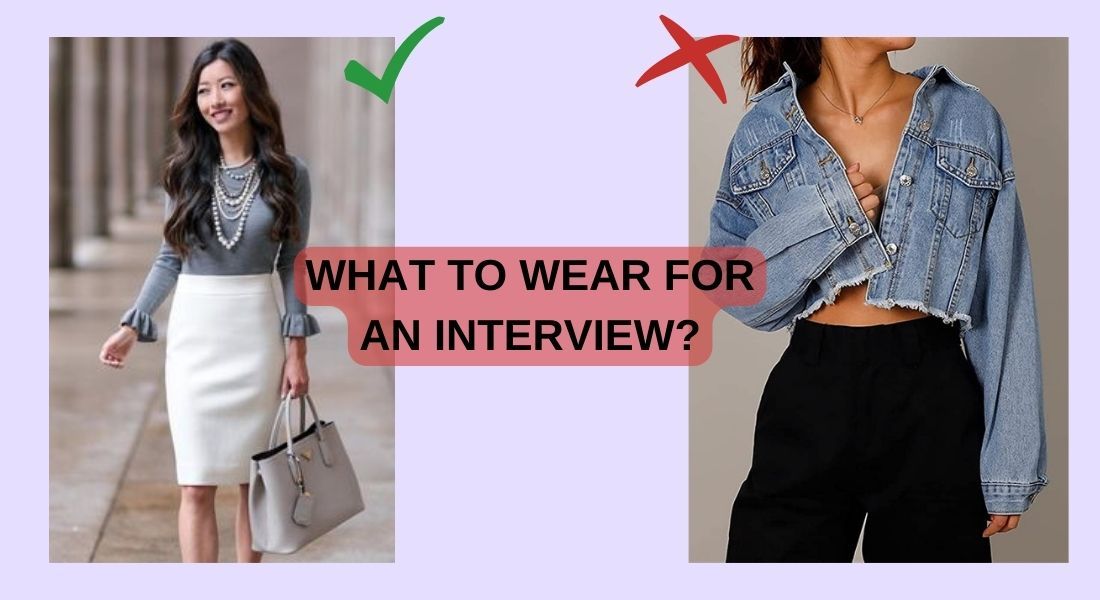The image serves as a "what to wear for an interview" guide, prominently featuring a contrasting comparison between two women. At the center of the image, there's a pink translucent banner with black text that states, "What to wear for an interview?" 

On the left, a woman, who appears to be Asian, is impeccably dressed in professional attire. She sports a long brown hairstyle, and her outfit includes a gray blouse adorned with ruffled sleeves and layers of pearl necklaces. The blouse is neatly tucked into a knee-length white pencil skirt. She carries a neutral grayish-beige handbag. A green checkmark in the upper right corner of this segment indicates her attire as appropriate for an interview.

On the right, the image shows another woman cut off at the chin, making her head indiscernible. She is dressed in a casual and unsuitable manner for an interview, wearing a cut off blue jean jacket with no shirt underneath, revealing her midriff. This jacket is paired with black pants. A red X in the upper left corner marks her outfit as inappropriate for professional settings.